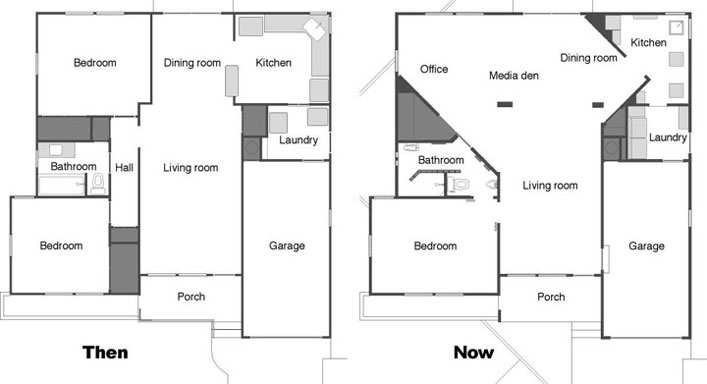This image features two detailed floor plans of a house, illustrating its evolution over time. The floor plan on the left, labeled "Then," begins with a bedroom in the upper left-hand corner. Moving to the right, there is a dining room followed by a kitchen. Below the bedroom is a bathroom connected to a hallway, and beneath the bathroom is another bedroom. Continuing rightward under the dining room is a spacious living room area that extends to a porch below. Under the kitchen, the layout includes a laundry room and a large garage at the bottom.

The second floor plan on the right, labeled "Now," showcases a modernized layout. The top left has been transformed into an open-concept space that includes an office, media den, dining room, and a living room extending downward. Adjacent to the living room on the bottom left is a bathroom with a bedroom located directly below it. The porch area remains situated under the living room. In the top right, the kitchen area has been downsized, with the laundry room still located beneath it. The garage remains in its original position, underneath the laundry room.